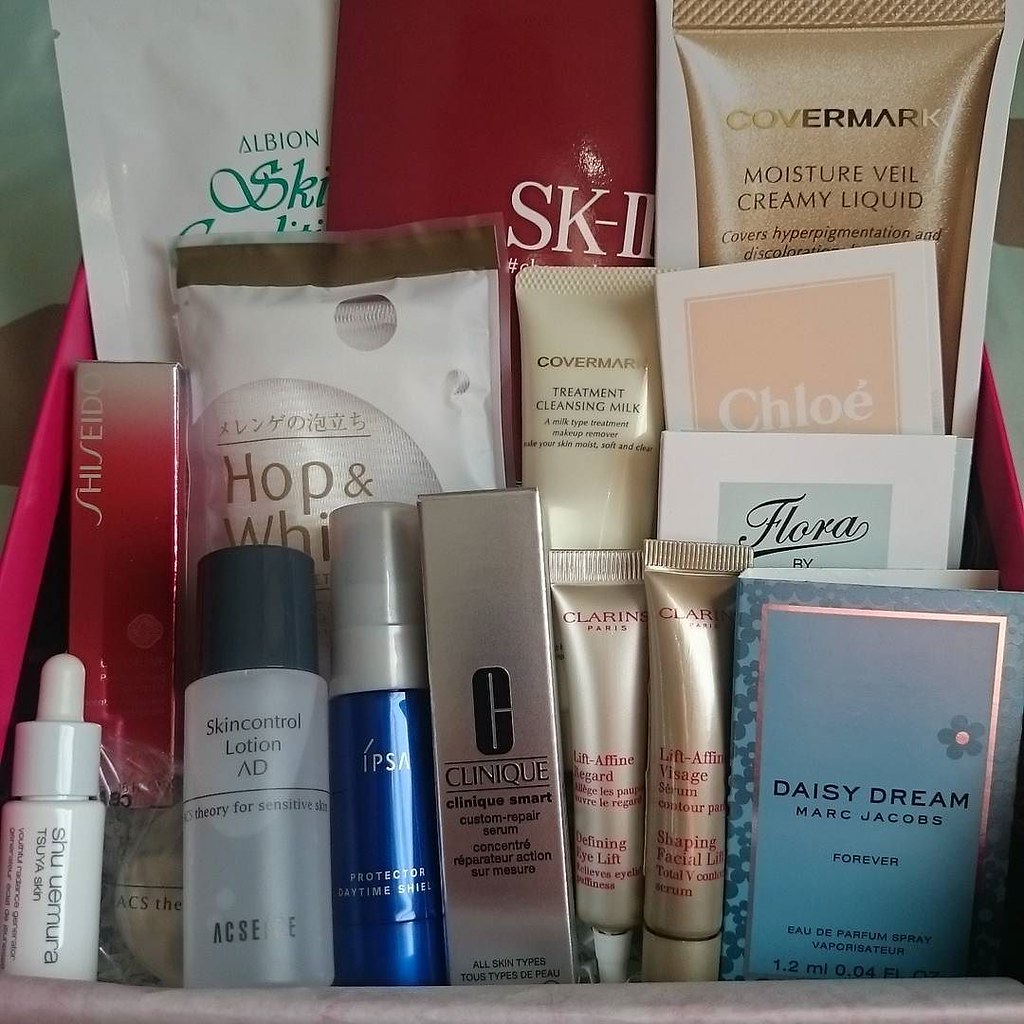The photograph showcases an organized collection of various makeup products thoughtfully arranged in a box with a visible pink rim along the left and right sides. The box is set against a dimly lit, shadowy white background that carries a subtle bluish tint. The arrangement of items within the box begins at the bottom left with a small white squeeze bottle labeled "Shu Uemura Tsuya Skin." Continuing to the right, there is a translucent plastic bottle with black text reading "Skin Controlled Lotion AD CS Theory for Sensitive Skin." Next in line is a blue bottle with a white cap, inscribed with the white text "IPSA Protector Daytime Shields."

Following this, the array includes a silvery box emblazoned with black text that says "C Clinique Clinique Smart Custom Repair Serum," with an additional description in French indicating it is suitable for all skin types. Two metallic squeeze bottles with gradations from silver to brass come next; one features a white pointed cap and the text "Defining Eyelift Relieves Eyelid Puffiness," while the other has a gold round cap and reads "Shaping Facial Lift Total V Something Scrum," both accompanied by French translations from Clarins Paris.

At the far right end of the row is a blue box marked "Daisy Dream" in black text, signifying it as a Marc Jacobs Forever Eau de Parfum Spray. Various other unidentified items can be glimpsed arranged behind these prominently displayed products, adding depth to the composition.